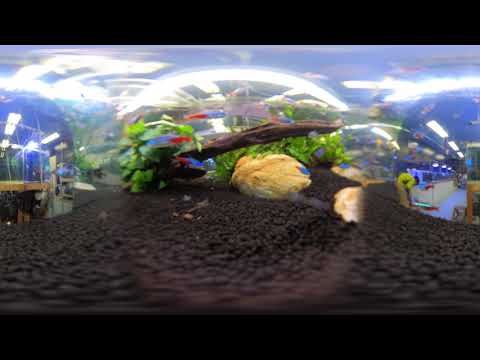This image depicts a highly distorted 360-degree view from inside a glass aquarium with low resolution, giving a sense that it's seen through VR goggles or similar tech. The aquarium contains black gravel on the bottom, a tan rock, and several green leafy plants. Small blue and red fish, about a dozen, are swimming around, initially blending into the background due to the image quality. The scene is set inside a pet or fish store, recognizable by the presence of multiple aquariums visible in the blurred background along with brown shelving units and silver railings. The ceiling is blue with overhead lights, suggesting indoor lighting. The vantage captures a store full of other tanks and enclosures, providing a more immersive feel of being inside the store itself.